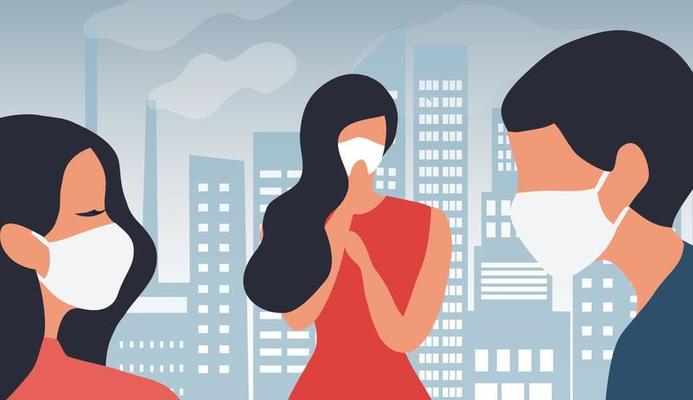This character poster presents a simplistic, vector-style illustration set in an urban environment with a cityscape backdrop, including faintly depicted skyscrapers and smoke stacks emitting white puffs of smoke. The artwork, featuring three cartoon figures with a light tan complexion and identical white face masks, vividly captures attention. Positioned on the left is a woman in a pink top, shown from a side profile with her black hair pulled behind her ear. In the middle stands another woman, waist-up, wearing a bright red dress; her long wavy black hair drapes past her elbow to her left, and she has one hand near her mask-covered mouth. On the right is a male figure in a teal blue shirt, also depicted in a side profile. Notably, the male and the woman in the middle lack visible eyes, while the woman on the left has a clear eye. The backdrop buildings feature a navy blue hue with white rectangular windows, emphasizing the industrial city scenery.